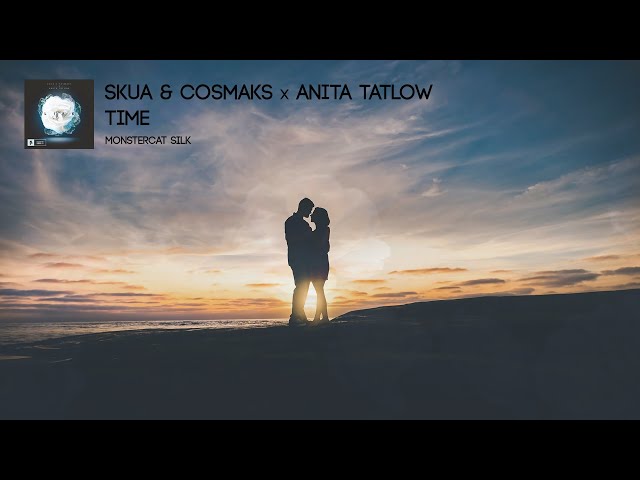This image appears to be a digital media recording cover for a music release. It depicts a silhouette of a man and woman standing close, looking into each other’s eyes with the setting sun between them, along what seems to be a beach with the sun low on the horizon. The sky is a gradient of blues at the top, blending into yellows and oranges near the sun, with a few scattered clouds. The composition is primarily dark due to the backlighting, creating stark silhouettes of the couple. On the top left corner of the image, there is a square that likely features the album cover, displaying an image that resembles a white rose or flower. Above the couple, the text reads "Sukua and Cosmax X Anita Tatlow," with the song title "Time" and the album name "Monstercat Silk" indicated beneath it. The photo captures a romantic and serene moment, with the panoramic landscape adding to the overall emotive atmosphere.